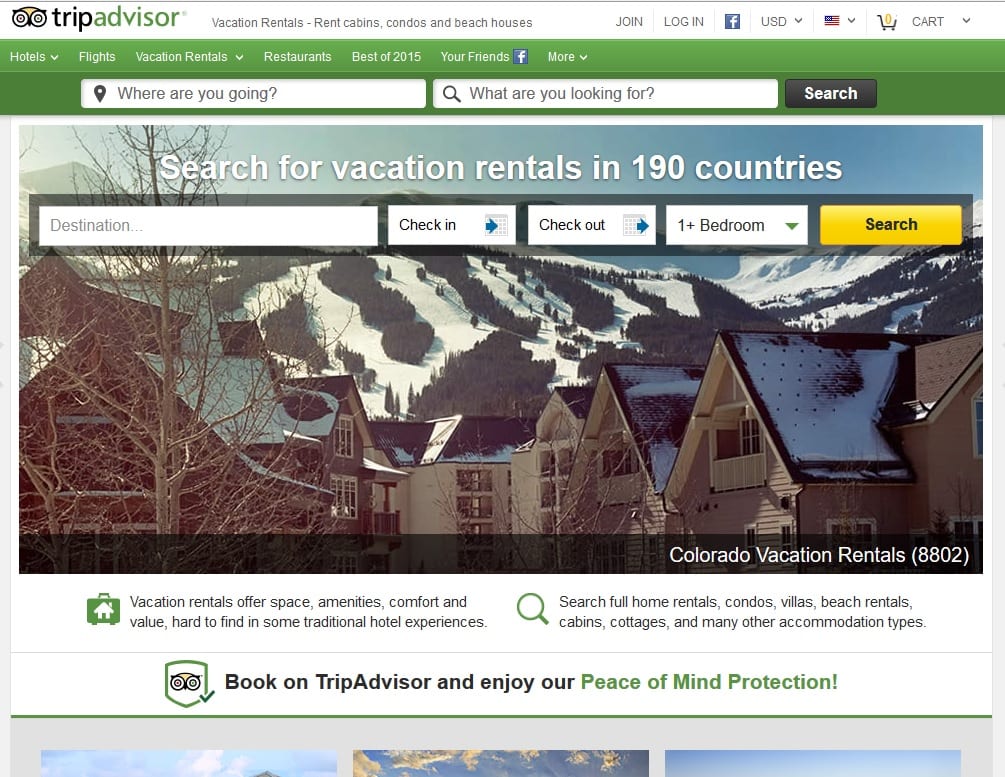This detailed screenshot from the TripAdvisor website features a myriad of elements organized for a potential traveler's convenience. At the top-left corner, the TripAdvisor logo is prominently displayed with the word "Trip" in black and "Advisor" in green, accompanied by an iconic owl illustration to its left. The website offers several features visible in the upper section, including options for "Vacation Rentals", and a tagline encouraging users to "Rent Cabins, Condos, and Beach Houses". 

On the right side of the header, users are presented with options to "Join" or "Log In", alongside icons for a Facebook login, currency selection (USD), an American flag, and a shopping cart indicating zero items.

Beneath this is a green navigation bar with tabs labeled "Hotels", "Flights", "Vacation Rentals", "Restaurants", "Best of 2015", "Your Friends", a Facebook logo, and more options, providing easy access to different sections of the site. 

A dual search bar is available below the navigation, with a primary location search prompt asking "Where are you going?" and a secondary search bar asking "What are you looking for?", followed by a black search button to the right.

The main content area features a large promotional image captioned "Search for Vacation Rentals in 190 countries", showcasing a picturesque snowy residential area. The houses are white with black roofs lightly dusted with snow, set against a backdrop of snow-capped mountains and surrounded by snowy fields. 

Below the image are form fields for users to input their desired destination, check-in and check-out dates, and bedroom preferences, functioning as filters for refining vacation rental searches. The image caption specifies "Colorado Vacation Rentals 8802".

The overall color scheme of the website is predominantly green and white, consistent with TripAdvisor's branding.